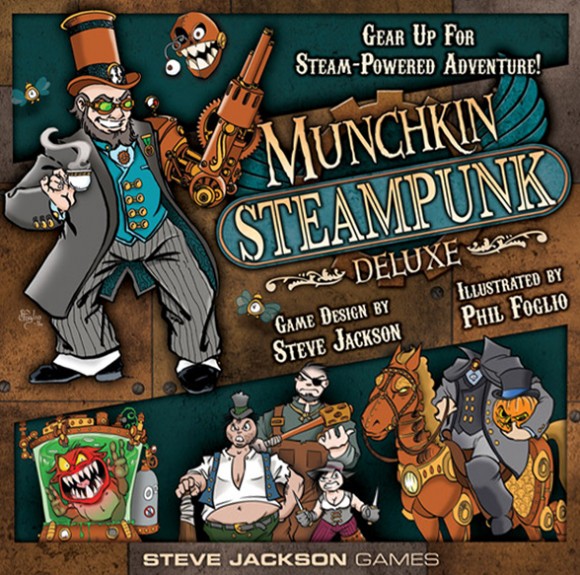The cover image is for a board game titled "Munchkin Steampunk Deluxe," designed by Steve Jackson and illustrated by Thiel Foglio. The cover features vibrant, hand-drawn illustrations, emphasizing a steampunk theme. At the very top left corner, there's a detailed character resembling the Mad Hatter from Alice in Wonderland. This character is dressed in pinstriped gray pants, black and white boots, and a black business coat with a blue vest underneath, adorned with golden buttons. He wears a large brown top hat with a clock on the front and green goggles. His left arm is a mechanical, steampunk gun covered in bronze cogs, while his right hand holds a steaming teacup. 

Next to this character, in the top right corner, white text reads, "Gear up for steam-powered adventure!" Below it, the game's title, "Munchkin Steampunk Deluxe," is written diagonally in gold with a blue background and flanked by blue wings. 

The bottom center of the cover features the text "Steve Jackson Games." Surrounding these central figures are numerous additional cartoon-style characters and elements. These include a jagged machine with white eyeballs on springs, a headless horseman riding a sinister peridot-eyed brown horse with yellow plating, and various other whimsical figures such as a small woman holding two swords and a man in overalls wielding a honeycomb-patterned club. Another notable figure wears a white tank top, a corset, pinkish pants, and a top hat, while yet another character, appearing to be an enemy, has a large belly, green pants, a brown wooden club, and black belt. 

Detailed and eclectic, the cover's illustrations convey an adventurous and imaginative steampunk universe designed to captivate the viewer's curiosity.